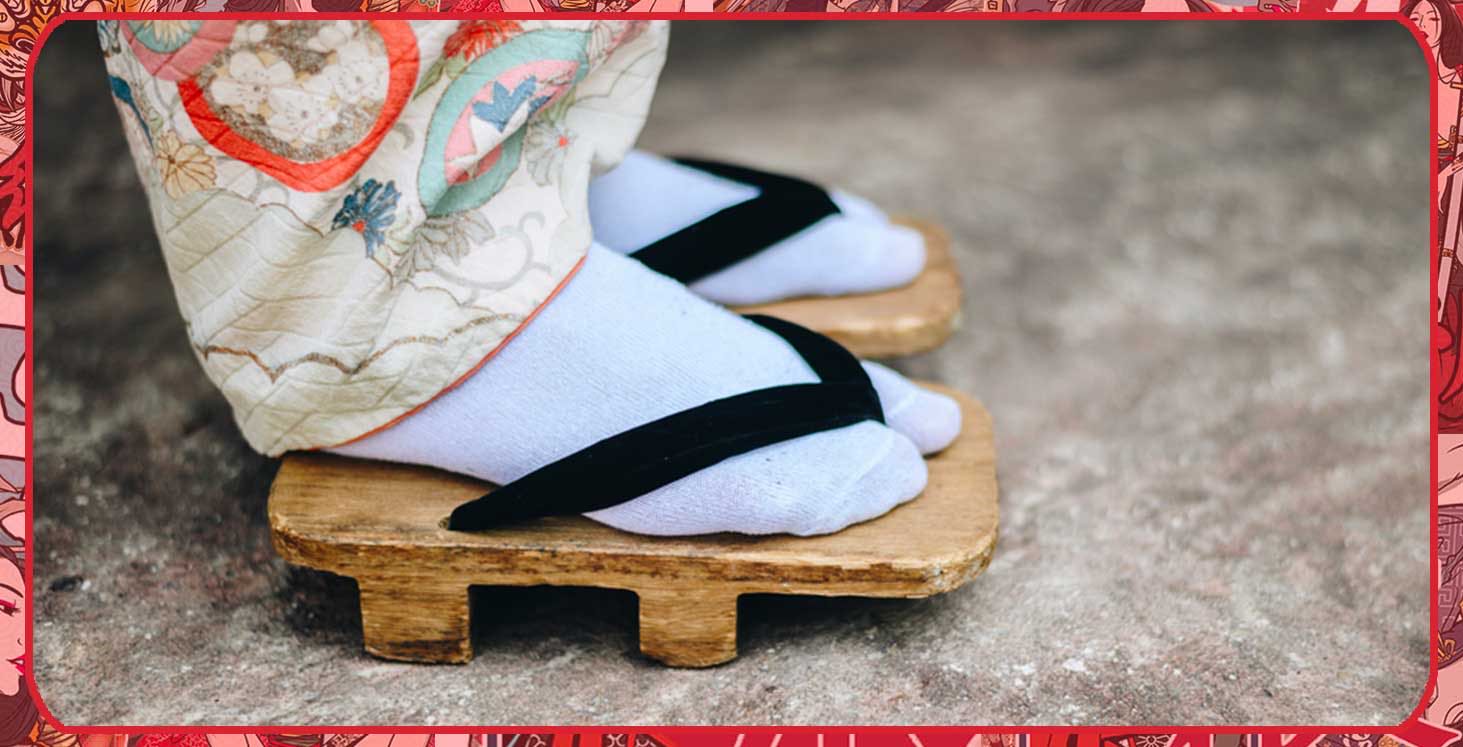The photograph captures an outdoor scene focused on the feet of a woman standing on a gray stone surface, likely concrete. Her attire includes loose-fitting pants or a dress adorned with a beige backdrop and floral print. She is wearing traditional Japanese wooden sandals, known as geta, which feature wooden soles and black straps that go between her toes. The woman also wears white socks with these sandals. Surrounding the image is a predominantly red border decorated with comic book-style illustrations of women's faces, specifically including women with brown hair in the top right and bottom left corners. These details suggest a blended artistic tribute, integrating elements of traditional Japanese culture and modern visual art styles.